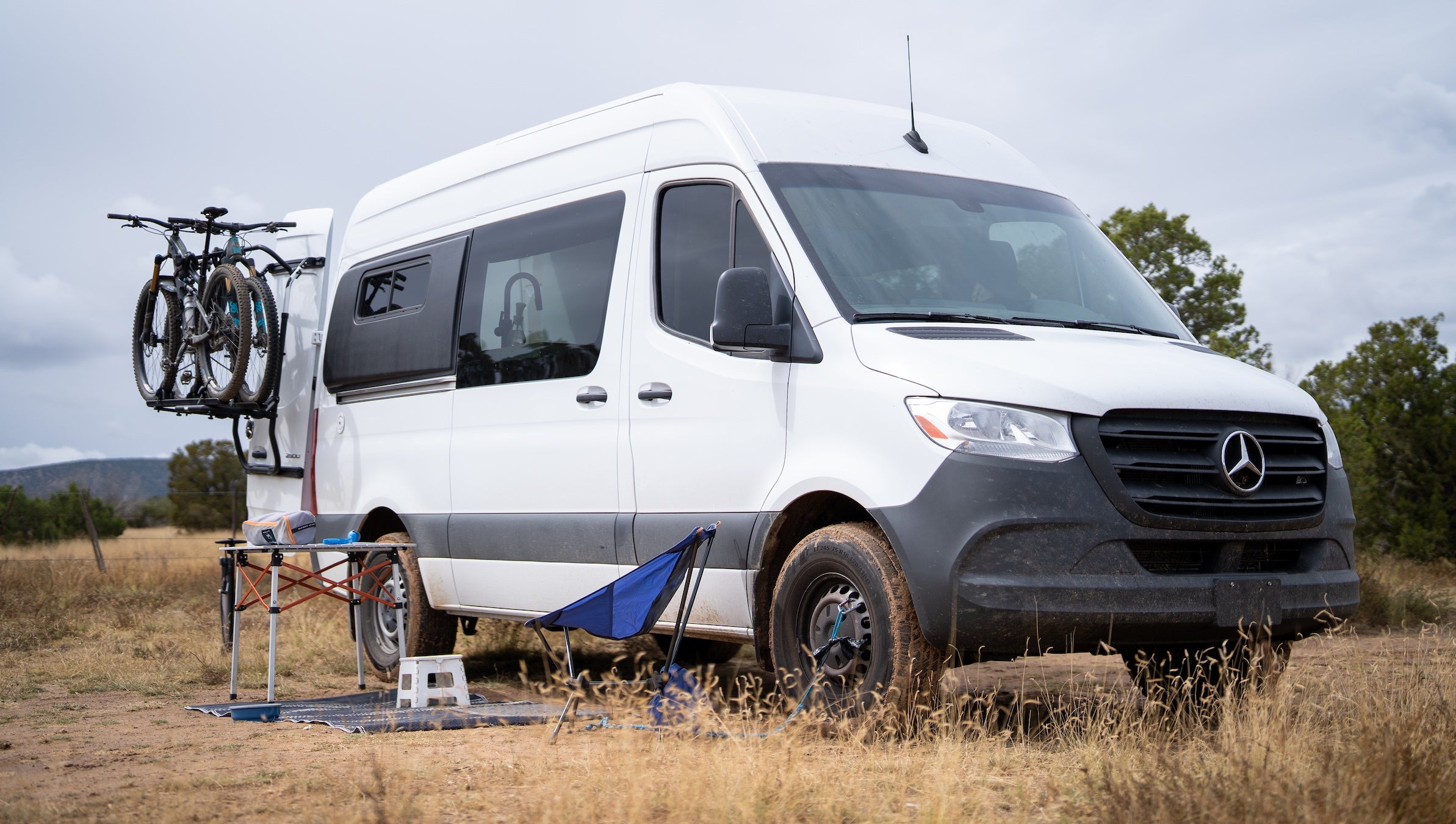A daytime photograph showcases a white Mercedes camper van parked in a field of dry, brown grass. The van, which has its back doors swung open, features three folded bicycles attached to a rack on the rear door. The vehicle’s tires display traces of mud, and the windows are tinted. Set up beside the van are a blue camping chair with a white footstool placed in front of it, a small camp table, and another piece of equipment that resembles a mat. The setting is dotted with several trees visible over the hood and in the background, contributing to the somewhat overcast ambiance of the scene, with the sky being a mix of blue and gray clouds.